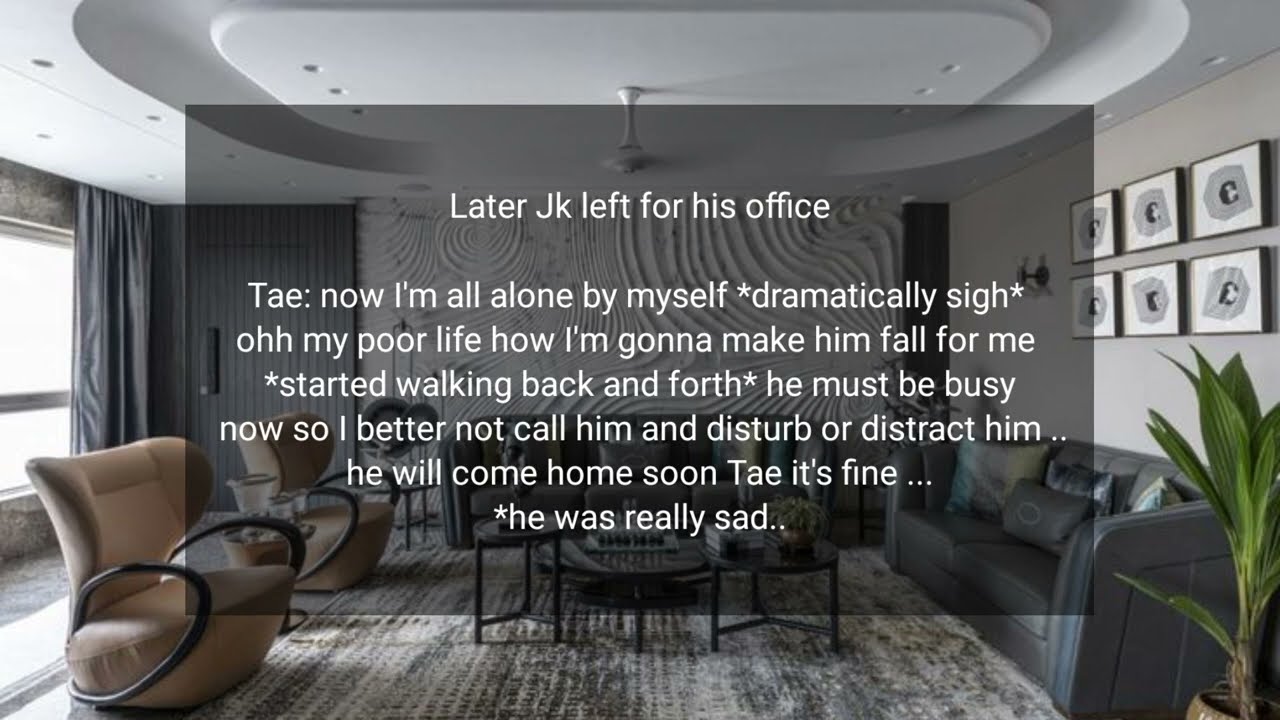This is a horizontal rectangular image depicting a slightly futuristic-looking living room. The ceiling is white with a circular design featuring notches, which give it a somewhat unreal, almost plastic or rubber-like appearance. A modern-looking light fixture hangs from the center of the ceiling. On the right side of the room, a gray wall showcases two rows of three pictures each. Below these pictures, there is a gray leather couch adorned with pillows. In the lower right-hand corner, a plant can be seen resting on the floor.

The center of the room is dominated by a large area rug with a table placed in the middle. On the left side, there are two brown chairs with high backs and black oval armrests, which provide an interesting contrast. Behind these chairs, a window draped with gray curtains lets in some natural light.

Superimposed over the image is a light gray text box with white lettering, formatted centrally in about six or seven lines. The text reads: "Later, JK left for his office. Tay, now I'm all alone by myself, dramatically sigh. Oh, my poor life, how am I going to make him fall for me. Started walking back and forth. He must be busy now, so I better not call him and disturb or distract him. He will come home soon, Tay. It's fine. He was really sad." This text suggests a scene from a romantic story, featuring a character named Tay expressing loneliness and longing after JK has left for his office.